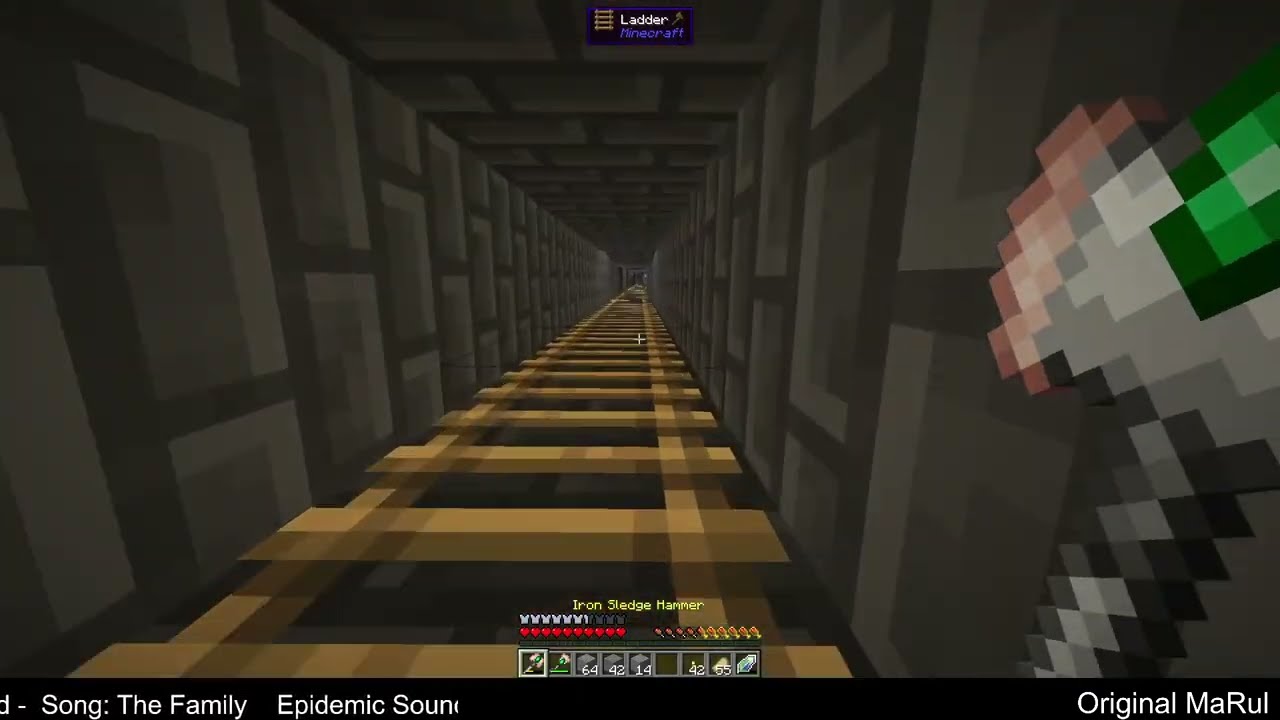The image is a detailed screenshot of a Minecraft game. It depicts a character climbing a long ladder that stretches from the bottom of the view to the top, above the center, disappearing into the distance. The ladder is set against dark gray and black stone walls that form a tall, narrow hallway. The floor appears to have varying shades of brown, tan, and black, creating a stair-like visual effect. In the upper portion of the screen, the word "Ladder" is displayed, emphasizing the character's current action. The character is holding an axe with an emerald gem embedded at the top; the axe has a silver-gray handle and a bladed end that is light brown in color. Below this, text reads "Iron Sledgehammer." At the bottom of the screen, a user interface showcases the character's status with an armor bar about two-thirds filled on the left and a health bar half-filled on the right. Additionally, a hotbar displays the character's inventory, including the Iron Sledgehammer, a flower, three blocks, empty slots, torches, paper, and an unidentified item. On the bottom left of the screen, text reads "Song: The Family, Epidemic Sound," indicating the current background music. In the lower right, the phrase "Original Maruul" appears, with the 'M' and 'R' capitalized.